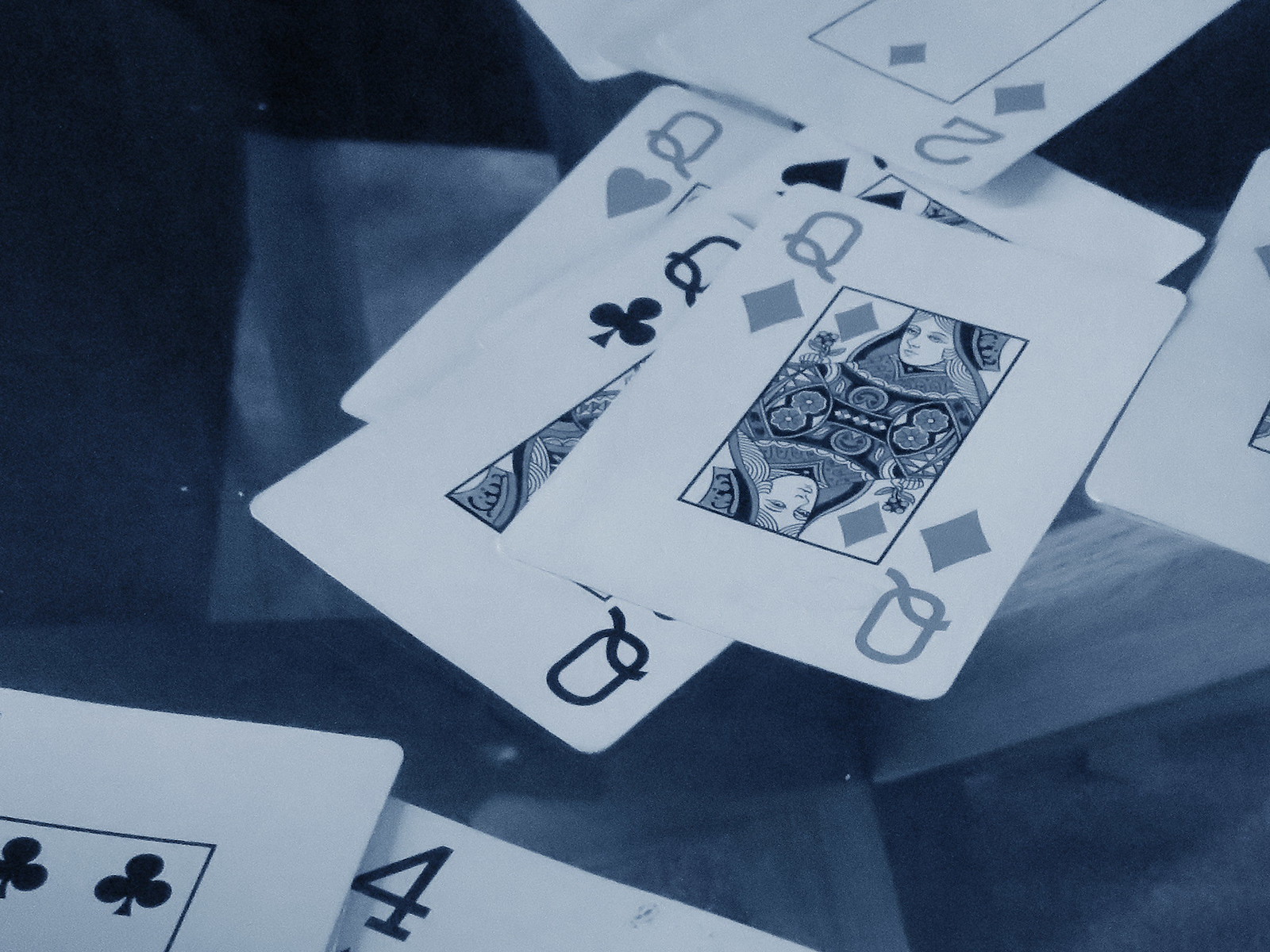The image showcases a collection of playing cards arranged artfully on a wooden surface. The four queens—the Queen of Diamonds, Queen of Clubs, Queen of Spades, and Queen of Hearts—are prominently positioned together, each tilted at various angles. The cards are presented in black and white, rendering the traditionally red Diamonds and Hearts in shades of gray, while the Clubs and Spades remain in black. At the top of the image, the Two of Diamonds is visible, positioned upside down. Near the bottom, there is an unidentifiable card from the Clubs suit and a separate card displaying the number Four. The wooden surface on which the cards rest has a varied grain pattern, with sections that are both light and dark, adding depth and texture to the monochromatic composition.